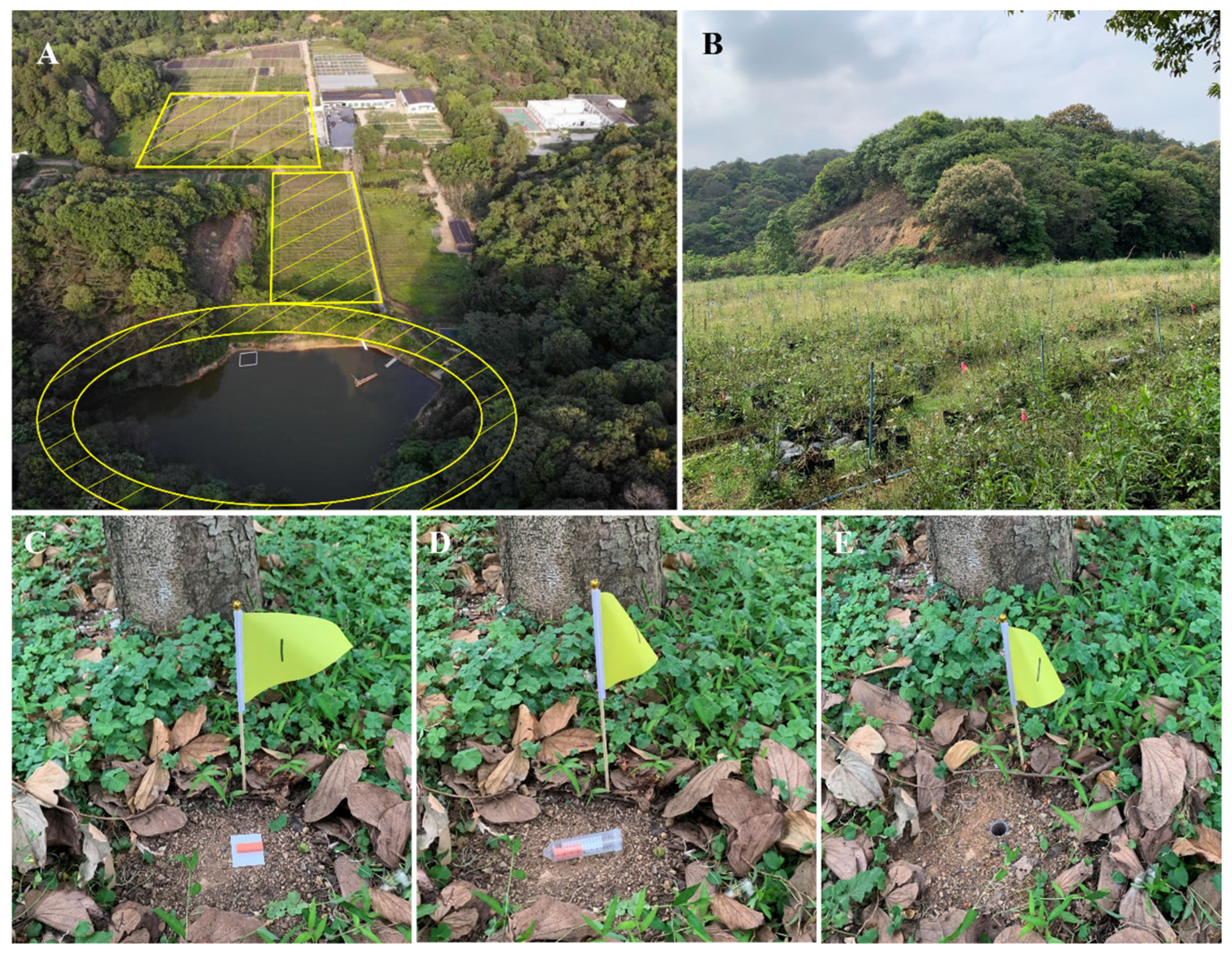The image is a composite of five labeled sections, A through E. The overall layout is a rectangle divided horizontally, with the top half consisting of two parts and the bottom half of three parts. 

In the top left corner, Picture A features an aerial view of a landscape showcasing a square, rectangle, and circular track highlighted in yellow with diagonal bars, amidst various trees and buildings. The top right corner, Picture B, presents a ground-level view of the same location, under an overcast sky. It shows a mound of dirt overgrown with trees and plants, along with two small red flags.

Occupying the bottom half, Picture C (left-most) displays a close-up of a tree with a yellow flag labeled "1" planted at its base, next to something orange and white, perhaps a soil sample indicator. Picture D (middle) similarly shows the same tree and flag, but with an orange substance inside a nearby tube. Finally, Picture E (right-most) depicts the same scene with the tree and flag, now featuring a hole in the ground, suggesting a sample had been taken.

Overall, the sequence highlights a process of marking, sampling, and examining a specific plot of land across the series of images.